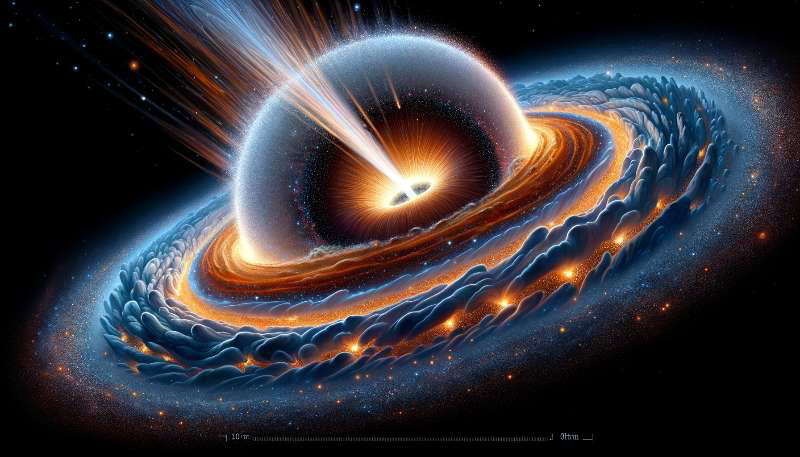This striking, graphically designed image captures a celestial object in the depths of outer space. It features a landscape-oriented canvas dominated by a high-contrast scene with a dark black background, indicative of the vast universe, peppered with small, glowing dots of red, white, and light blue, signifying distant stars or planets. At the heart of the image lies a large, central sphere, possibly a planet, enveloped in a dramatic burst of light emanating from its core. Surrounding this sphere are multicolored rings of orange, blue, and light gray, which alternate in softness and gradually dissipate into a dust-like material at their edges. These rings, seeming to spiral outward, contribute to a nebula-like effect, with dark orange and gray clouds adorned with tiny white crests. The central element appears almost like a floating egg, with a blazing hot white and red core projecting a radiant beam of light, encapsulated by blue, cloud-like formations studded with tiny yellow specks, creating an ethereal, starburst phenomenon.